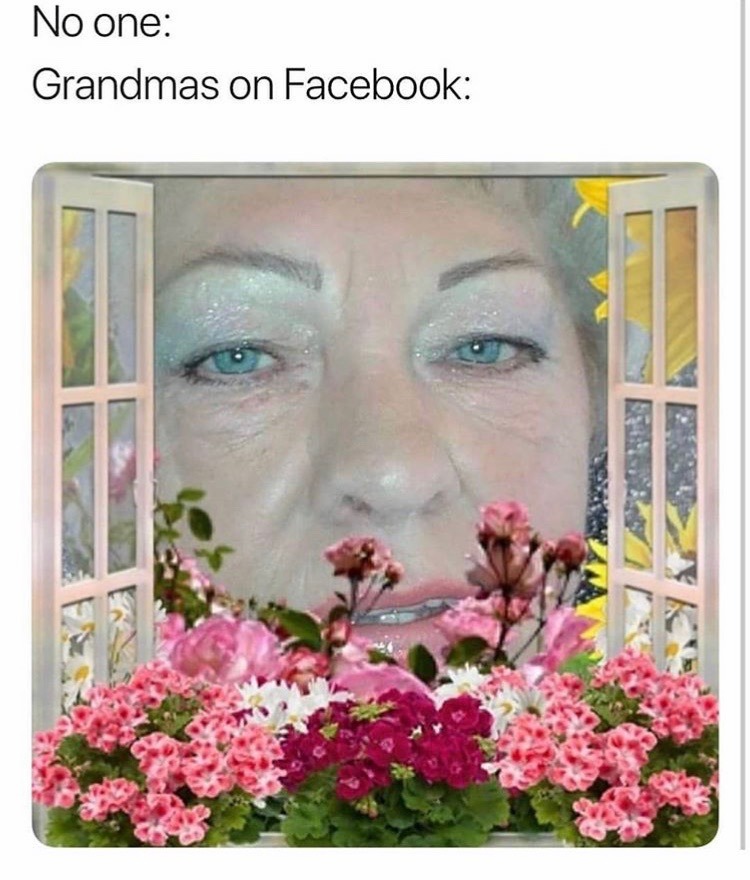In this image, we see a close-up of an elderly woman's face peering through open glass doors, reminiscent of the inside of a dollhouse. Taking up most of the frame, her face is in sharp focus, emphasizing her gray eyes and weathered, yet gentle expression. Below her face, a flowerbed featuring a variety of flowers and greenery, meticulously detailed but clearly miniature, stretches across the doorway, adding a sense of whimsical scale. The text on the screen reads "No one," followed by "Grandmas on Facebook," humorously alluding to the scene. The colors in the image range from black, white, yellow, green, blue, light blue, purple, to pink, with different shades of gray. The words are positioned at the top, while the vivid image dominates the lower section. Overall, the setting and caption suggest a playful meme format typical of Facebook, cleverly showcasing the grandmother's appearance on the social media platform.